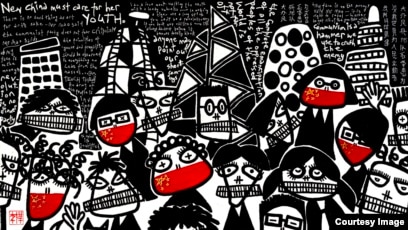The image is a black-and-white, cartoonish drawing reminiscent of Picasso's style featuring a grotesque and abstract cityscape with five buildings in the background. In the foreground, numerous stick-figure-like people with heads of various shapes—triangular, square, and round—are depicted. Each person has uniquely detailed eyes and uniformly drawn mouths filled with teeth, contributing to their unsettling appearance. Some individuals wear solid red masks covering their nose and mouth, resembling the Chinese flag. A small, barely legible text in the upper left corner includes the word "youth," suggesting a possible context. Overall, the scene is a surreal blend of artistic whimsy and unsettling detail.